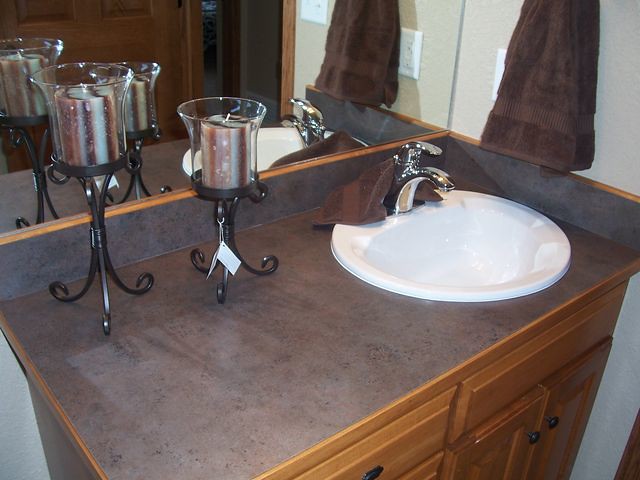The image is a color photograph of an unconventional bathroom vanity arrangement. The vanity, crafted from medium-tone wood, features a single round white sink situated on the right side rather than centered. The sleek chrome faucet, adorned with a single handle, has a brown washcloth draped over its back. 

To the right of the sink, just above the side splash, hangs a matching brown hand towel, suggesting a towel ring or bar is positioned slightly out of the frame. The countertop, resembling formica or slate, is complemented with a wood-tone trim along its edges, which extends to the top of the side and backsplash in a peculiar design choice. 

A frameless wall-mounted mirror reflects parts of the room, including light switches and a six-panel wood door, enhancing the bathroom's light and spatial perception. On the left side of the countertop, two wrought iron candle stands sit elegantly. Designed with curlicue feet and round faces, these stands hold clear glass candle holders with flared tops. Each holder encases a striped pillar candle with alternating hues of white, brown, and light brown. Notably, the shorter candle stand retains a price tag, indicative of recent staging or purchase.

The arrangement and décor come together to create a striking, albeit unusual, bathroom setting with a mix of mundane and curious elements.